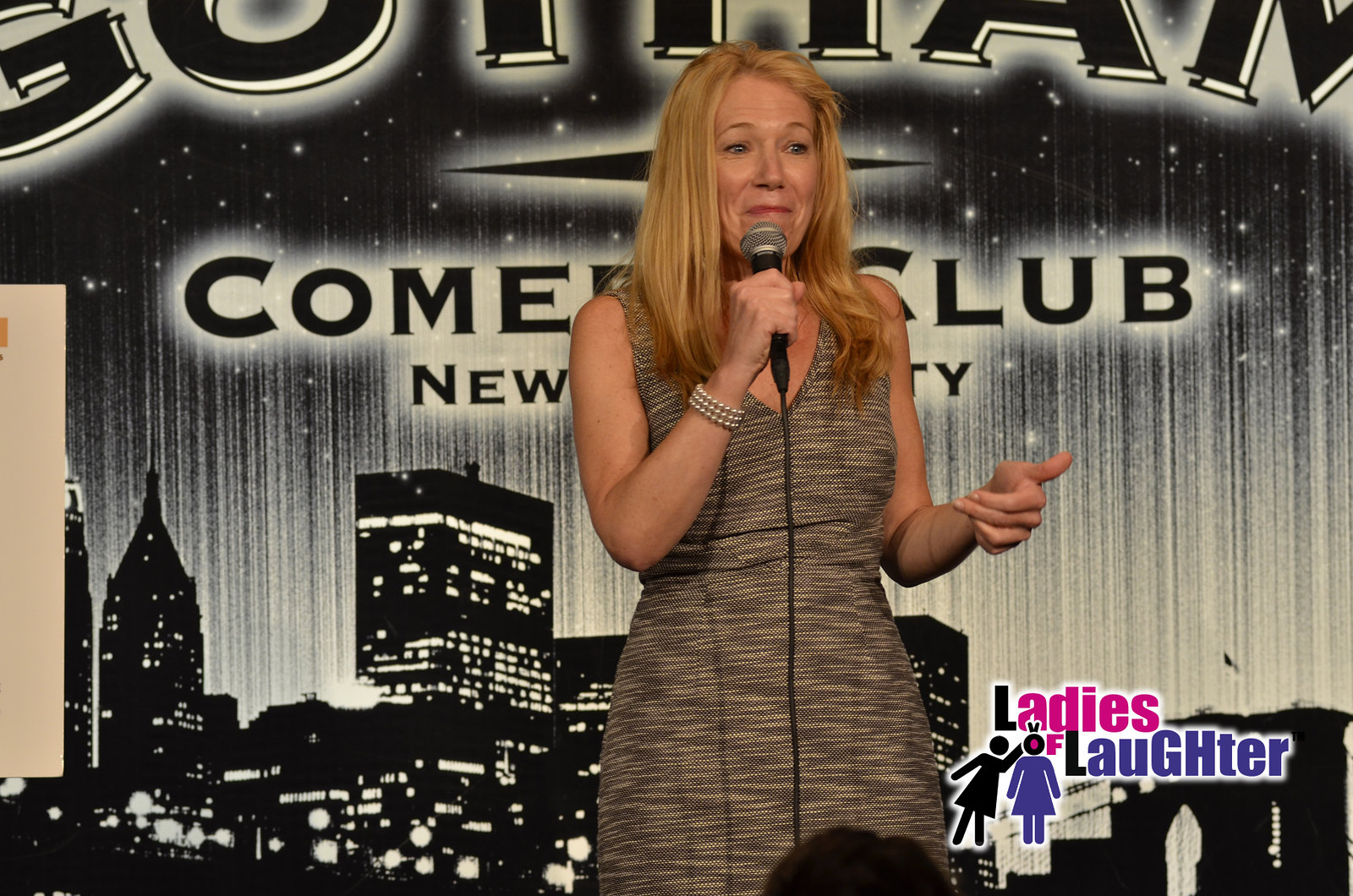The rectangular photograph captures a comedian standing on stage, set against an evocative black and white cityscape backdrop. The background depicts a night scene of a tall building skyline with illuminated windows, stars, and streaks of light reaching up into the dark sky. The partially visible signage above and behind her reads "Gotham Comedy Club, New York City," despite being partly obscured. The woman, likely in her late 40s or early 50s, is attired in a sleeveless, v-neck, black and white, or gray-striped dress. Her strawberry blonde hair frames her face, which bears a smirk, and she wears a pearl bracelet on her wrist. Holding a corded microphone to her mouth, she appears to be in mid-speech, with her other hand lifted halfway. The image's bottom displays an overlaid pink, purple, and black label, featuring the text "Ladies of Laughter" and outlines of two women resembling restroom door icons.